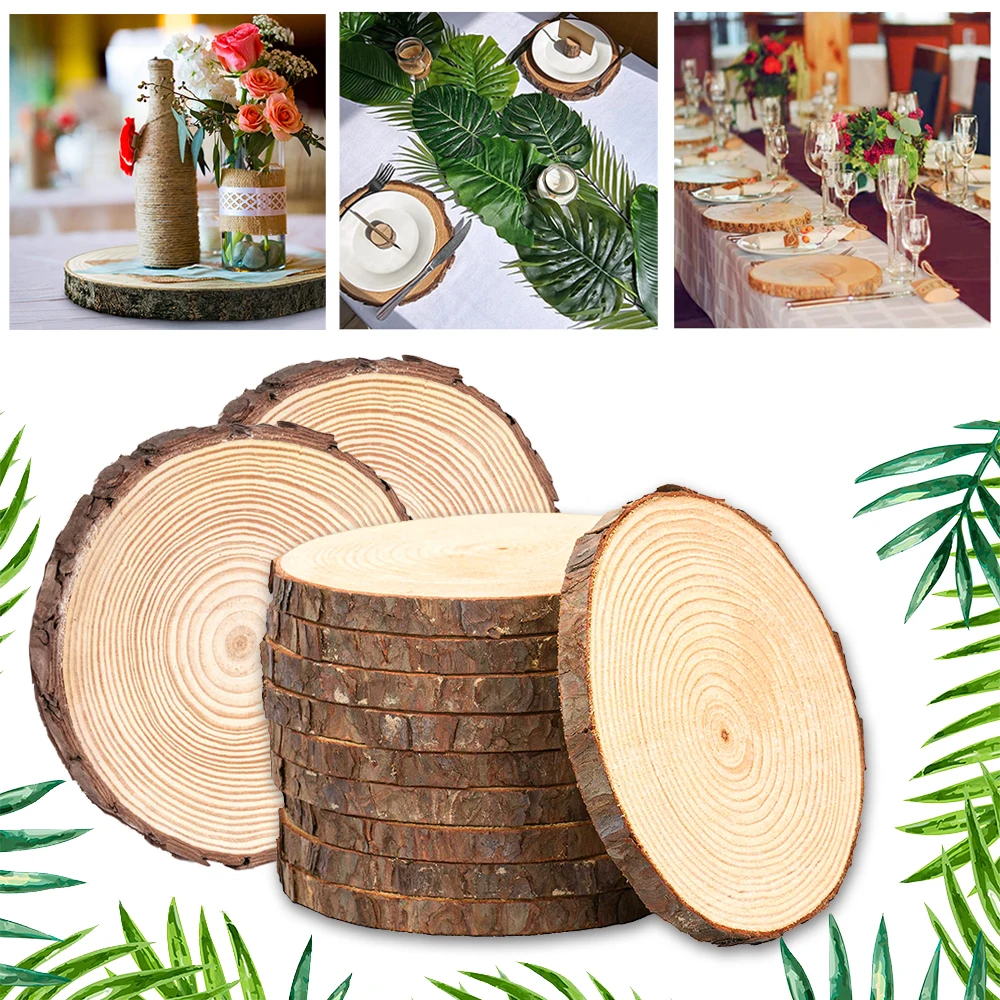The image is a composite of four photographs showcasing elegant rustic wedding reception decor, undoubtedly something that a wedding planner might feature on Instagram or Facebook. The bottom larger image highlights a stack of thinly cut wooden circles resembling tree trunks, with some laid against the stack. Above it are three smaller images, each depicting different aspects of the table settings. The first small photo captures a close-up of a round wooden cutout serving as a base for a centerpiece, which includes a glass bottle wrapped in twine and a jar adorned with burlap, filled with white flowers, baby's breath, and pink and peach roses. The middle image presents an overhead view of a table setup with white plates placed on similar wooden cutouts, accompanied by silverware and decorated with large green leaves and candles running down the center. The third image shows a long reception table with rows of wooden cutouts, white plates, clear glasses, and matching floral arrangements. The consistent theme of rustic wooden elements and green foliage ties the images together, creating a cohesive and charming wedding reception aesthetic.